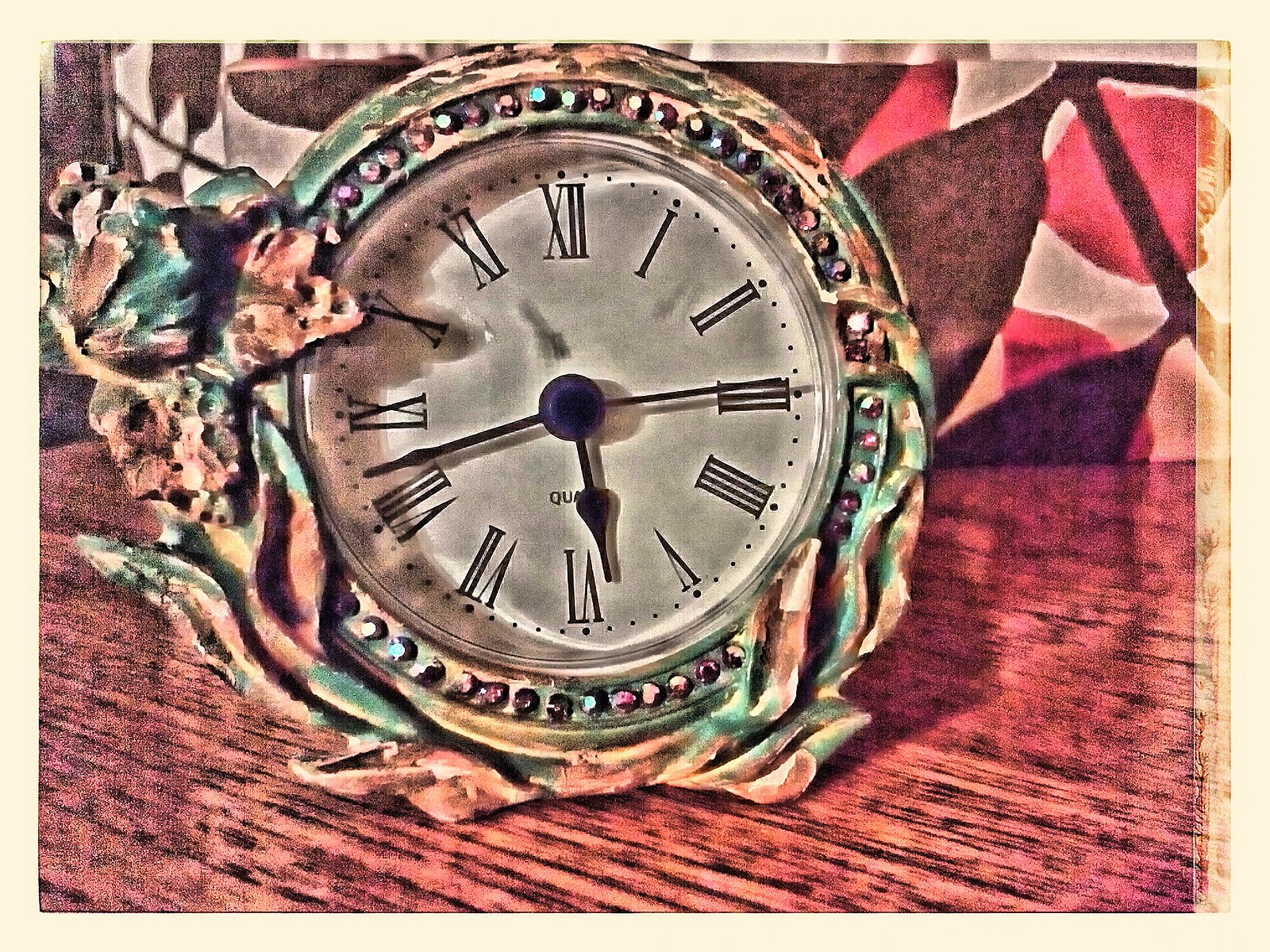The image is a detailed painting of a unique, rustic clock sitting on a wooden table with a distinct grainy texture. The circular clock face is adorned with tall, old-fashioned Roman numerals, with bold dots above each numeral and smaller dots in between, marking every 15 minutes. The hour hand points just before the six, the minute hand is between eight and nine, indicating around 42 minutes past, and the second hand rests at the three. The clock face is predominantly white, bordered by a silver circular frame. Surrounding this frame is a ring embedded with a variety of colorful gems including pink, orange, purple, blue, green, and white. This is followed by another circular border featuring a multicolored, watercolor-like floral design with discernible petals, stems, and leaves, particularly noticeable on the left side of the clock. The background fabric of the painting displays red splotches within a patterned design of pointy white areas, contributing to the overall artistic and textured appearance of the scene.